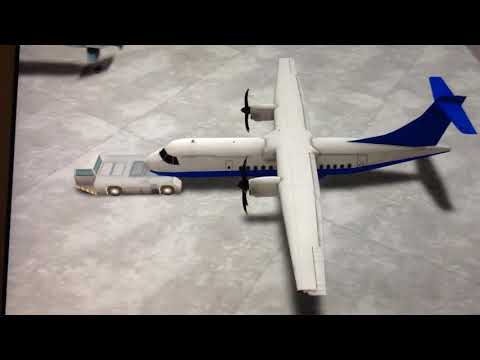The image, seemingly a high-angle shot rather than directly overhead, portrays what appears to be a 3D-rendered or possibly toy-like passenger propeller plane. The scene has an unusual texture, contributing to a somewhat surreal, animated feel. The plane, predominantly white with royal blue accents on its underbelly and tail, features black windows on the front and sides. It has two propeller engines, one on each wing, situated over the fuselage. The ground beneath the plane resembles large tiles, adding to the impression of its being a non-tangible model or rendering. The airplane is being tugged by a small white truck, akin to the tug carts seen at airports.